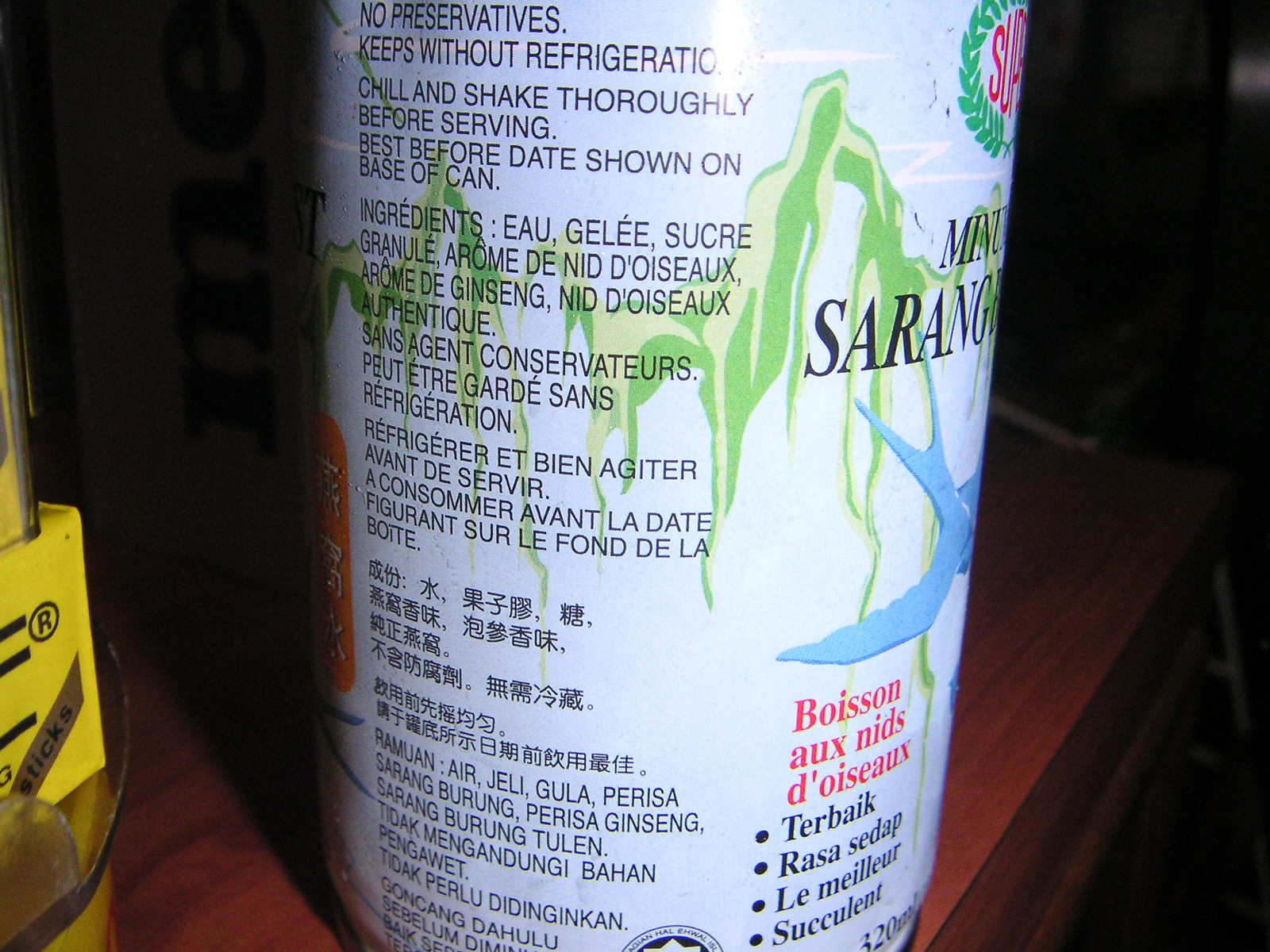This color photograph, in landscape format, captures a close-up view of a white beverage can adorned with green, blue, and red accents. The can prominently features black text at the top, stating "No preservatives, keeps without refrigeration. Chill and shake thoroughly before serving. Best before date shown on the base of can." The main text comprises foreign languages including French, with phrases such as "Eau gélée sucre granulé aromé de nid d'oissons" and "Boisson aux nids d'oissons," alongside Chinese characters.

The can appears to be from another country, with multilingual inscriptions and detailing. Although the photograph doesn't show the full top or bottom of the can, it does capture it from a side angle. The surface the can rests on appears to be a brown shell, and in the bottom left corner, a yellow object with silver rods and black lettering is visible. A blue object also occupies space to the right of the can. The image's overall background details and context further underscore its international essence, alluding to a unique beverage that transcends cultural boundaries.